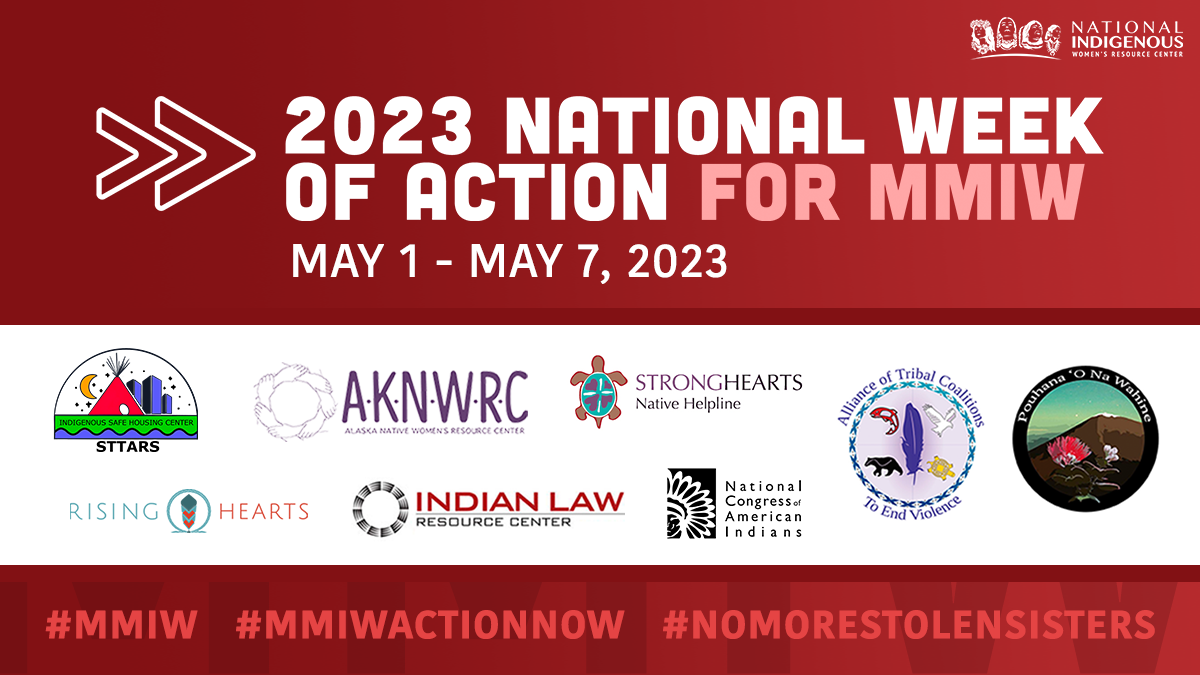The image is a detailed and informative poster advertising the 2023 National Week of Action for Missing and Murdered Indigenous Women (MMIW), taking place from May 1st to May 7th, 2023. The upper portion of the poster features a red background with prominent white text that reads: "2023 National Week of Action for MMIW, May 1st to May 7th, 2023." In the upper right corner, there is a logo for the National Indigenous Women's Resource Center. Below this, the background shifts to white, showcasing an array of logos from various supporting organizations, including the Indian Law Resource Center, Rising Hearts, National Congress of American Indians, Strong Hearts Native Helpline, and the Alliance of Tribal Coalitions to End Violence, among others. At the bottom of the poster, a red strip features hashtags in pink text, highlighting #MMIW, #MMIWActionNow, and #NoMoreStolenSisters. The overall design uses red and white as primary colors, with additional distinct colors in the organizational logos, effectively conveying the urgency and unity behind the cause.